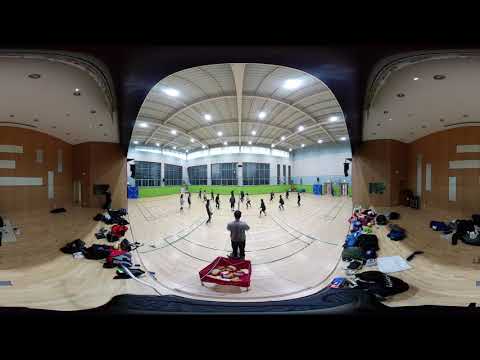The photograph, captured with a unique panoramic fisheye lens, provides a comprehensive, wide-angle view of an indoor school gymnasium. The image is divided into three distinct sections. In the central view, a man, possibly a referee, stands near a red table on the gym court, with a group of young children, seemingly around ten years old, positioned on the court. The children appear to be engaged in a game, their focus directed away from the man and towards the center of the gym, as though reacting to a volleyball or similar activity. The gym’s backdrop showcases numerous large windows, a gray wall, and multiple spotlights hanging from the gray ceiling. To the right, the background shifts to a green, blue, and gray wall, adjacent to a hallway visible through some windows. Surrounding the gym court on both sides are scattered personal belongings of the participants, including black bags, red backpacks, and jackets, strewn across the brown floor. The left side features a similar hallway with additional gear scattered about, further emphasizing the sense of activity and participation within the space. This comprehensive, multi-perspective shot vividly captures the dynamic environment and the organized chaos typical of a school gym setting.